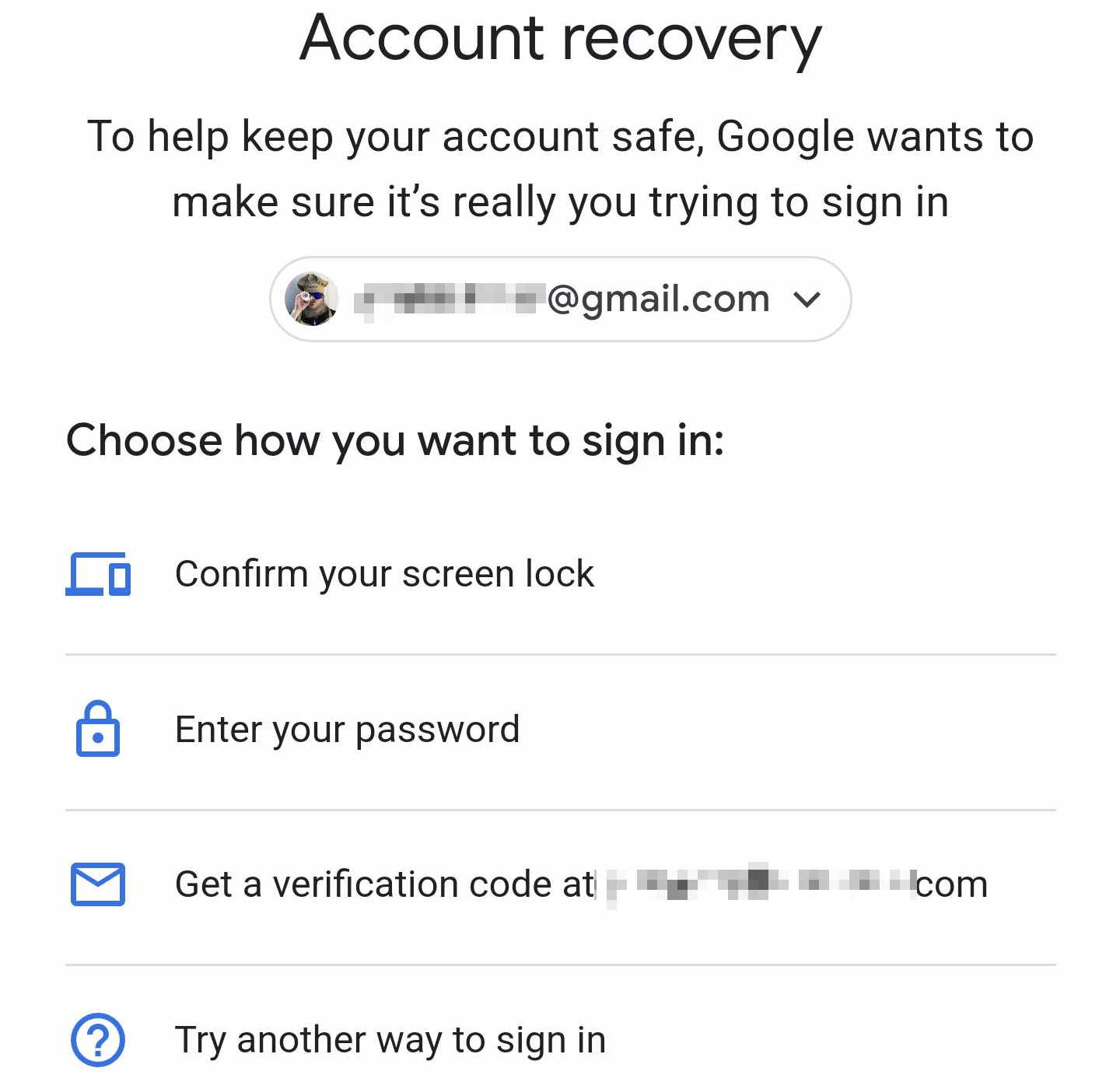In this instructional image, displayed against a white background, the title "Account Recovery" is prominently featured at the top center in bold black font. Beneath this header, within a gray elongated oval, the text reads, "To help keep your account safe, Google wants to make sure it's really you trying to sign in." 

The central section of the image includes a circle that might contain an image, possibly representing a user, although it's unclear due to pixelation. Adjacent to this is the partial email address, rendered as "*******@gmail.com," accompanied by a gray downward-pointing arrow.

Below this, in black font, it states, "Choose how you want to sign in..." followed by several options:
1. "Confirm your screen lock," depicted with a blue image resembling a smartphone screen.
2. "Enter your password," indicated by a blue padlock icon.
3. "Get a verification code at *******.com," accompanied by a blue envelope icon.
4. "Try another way to sign in," illustrated with a blue question mark inside a circle.

Each option is separated by a thin gray line, ensuring clarity and organization within the step-by-step instructional layout.